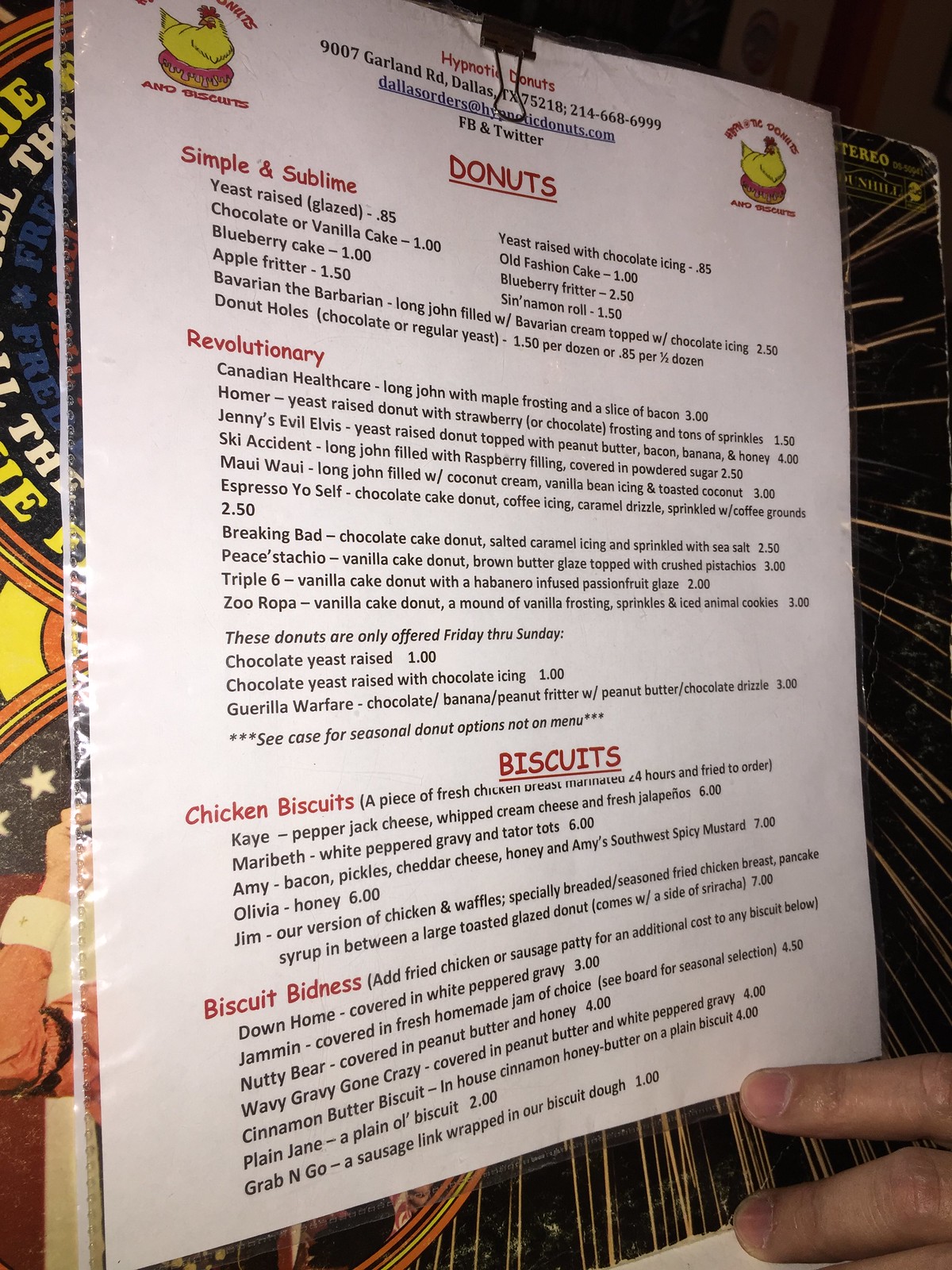In this image, we see a comprehensive menu from "Hypnotic Doughnuts and Biscuits" prominently displayed. The menu occupies nearly the entire image and appears to be a single-page layout. At the top, the title "Hypnotic Doughnuts" is centered, flanked by logos of a yellow chicken sitting on a glazed pink doughnut. Above the chicken's head, the text reads "Hypnotic Doughnuts" and below the doughnut, in a red font, it states "and Biscuits."

The menu is split into sections, roughly 60% dedicated to doughnuts and 40% to biscuits. The doughnut section features:

1. **Simple and Sublime**:
    - Yeast-Raised Glazed
    - Old-Fashioned Cake
    - Apple Fritter
    - Chocolate or Vanilla Cake

2. **Revolutionary**:
    - Canadian Health Care
    - Homer
    - Ski Accident

Each doughnut in the revolutionary section has custom names accompanied by detailed descriptions and prices.

The biscuit section includes:

1. **Chicken Biscuits**:
    - Various options with detailed toppings and fillings.

2. **Biscuit Bidness**:
    - Custom biscuits with unique flavors and combinations.

The menu is vibrant and appealing, promising a delightful array of inventive and traditional doughnut and biscuit options.